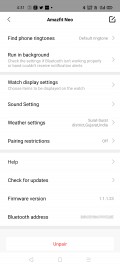A blurry, low-resolution image displays the settings page of an unidentified app, potentially related to Bluetooth configuration, given certain visible elements. The background is white with black text detailing various options such as "Phone," "Ringtones," "Run in Background," "Help," "Check for Updates," "Firmware Version," and "Bluetooth Address." Due to the image quality, many words are hard to decipher. A distinctive "Unpair" button, colored white with red letters, is situated at the bottom of the screen. The notification area of the phone is partially visible but equally unclear, with predominant black and white tones.